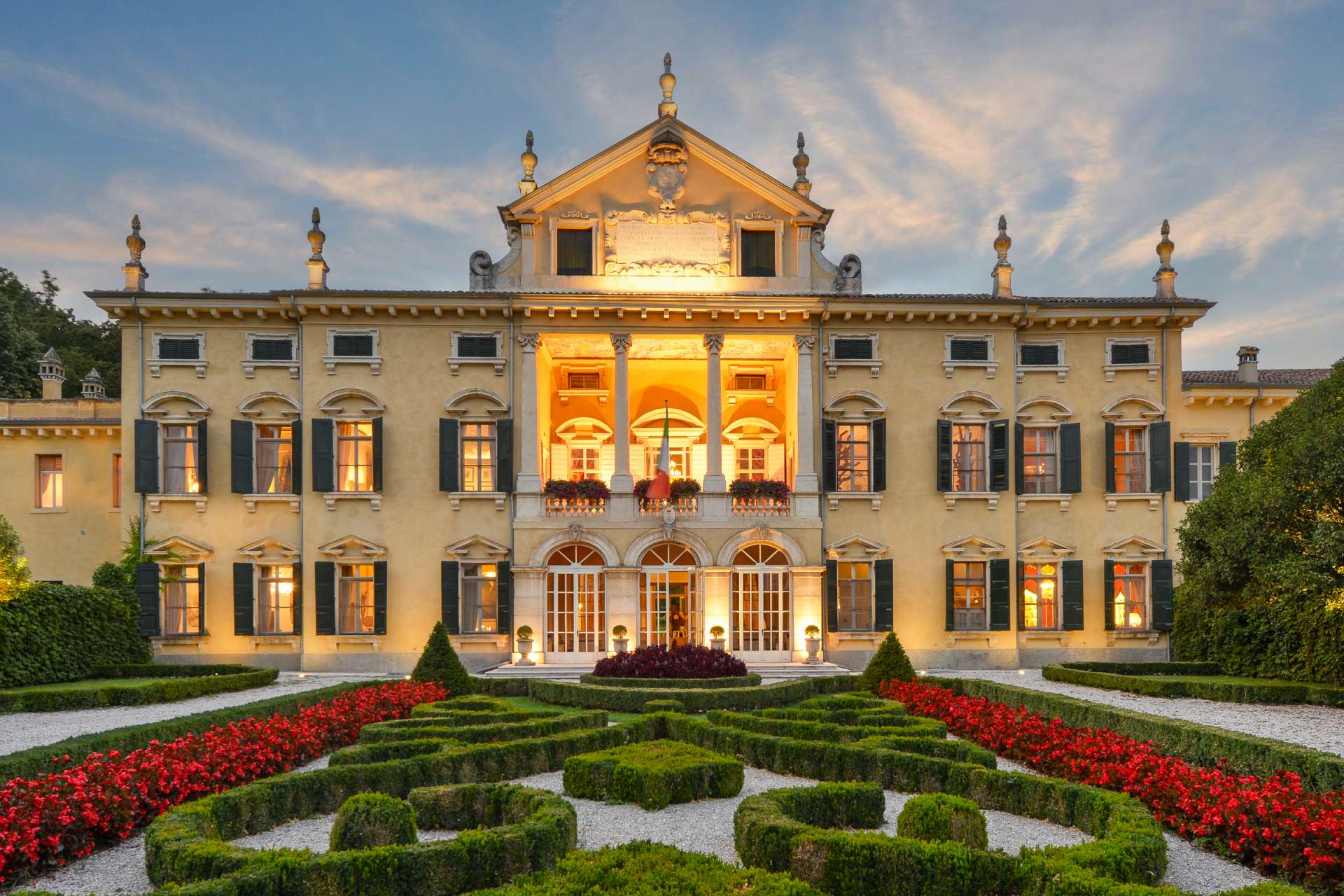The image showcases a sprawling, three-story mansion with a beige stucco exterior and dark shutters. Resembling an ornate hotel or a grand 17th-18th century manor, the building features a multitude of windows—approximately 30-40 in total—that are all illuminated. The upper floor boasts balconies rich with lush plants, and a prominent porch deck projects from the top. The mansion is framed by meticulously manicured gardens, including a low hedge maze with swirling patterns designed for leisurely walks and tastefully interspersed with vibrant red azaleas and flowers. On each side of the garden, concrete walkways lead up to the front steps, which are flanked by three grand entrance doors. The setting is serene, with a muted, bluish-white sky providing a tranquil backdrop.